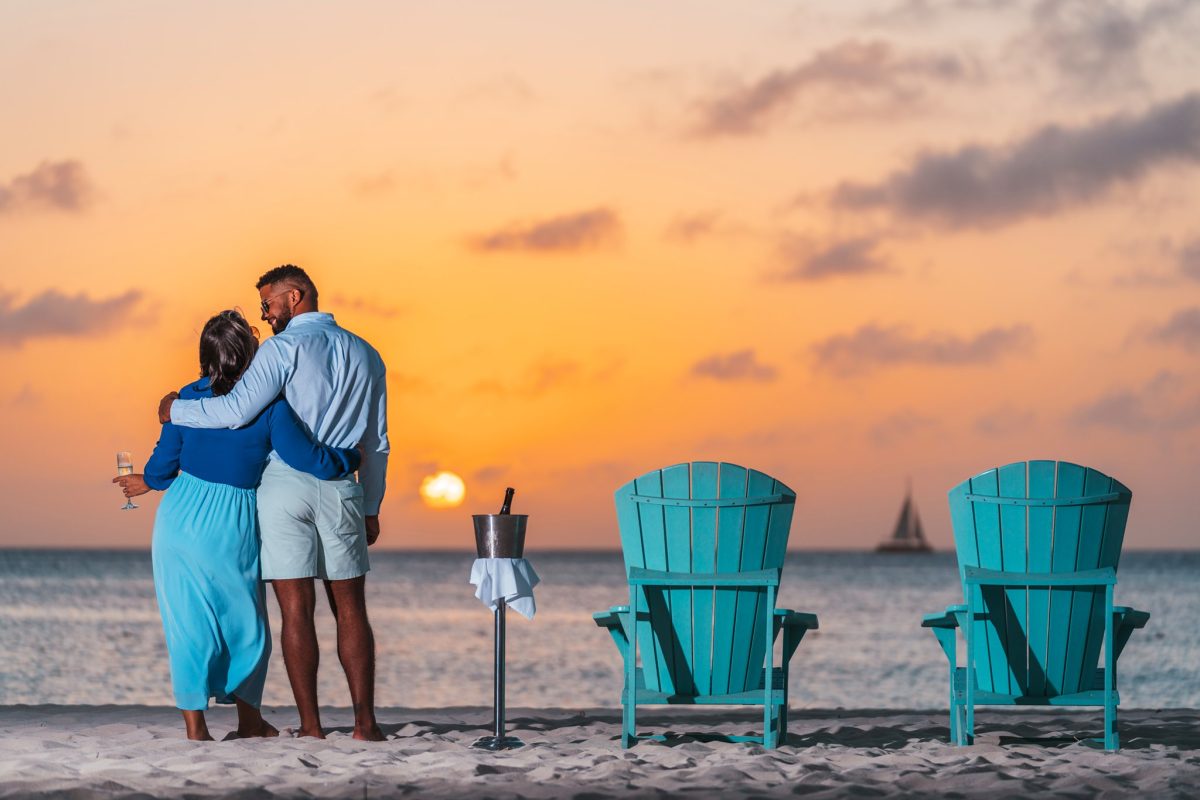A couple, deeply in love, embraces on a serene beach, gazing into each other's eyes with warm smiles. The woman, on the left, is adorned in a light blue skirt and a dark blue top, holding a glass of champagne in her left hand. Her blondish-brown hair cascades gently as she wraps her right arm around her partner's waist. The man, taller by six inches, stands to her right in a light blue button-down and light gray shorts, his left arm securely around her shoulders, his right arm relaxed at his side. His tan complexion, brown hair, and a well-groomed beard and mustache complement his attire. Next to them, a pedestal stands in the sand, holding a champagne bucket brimming with wine. Beyond this, two teal wooden beach chairs face the calming waters of the ocean, their backs hinting at a perfect spot to take in the view. In the distance, a sailboat cuts a blurry, serene figure on the horizon beneath the setting sun, casting beautiful pinks and oranges across the sky. The entire scene captures an intimate and idyllic moment, perfect for a romantic getaway brochure or a cherished personal memory.